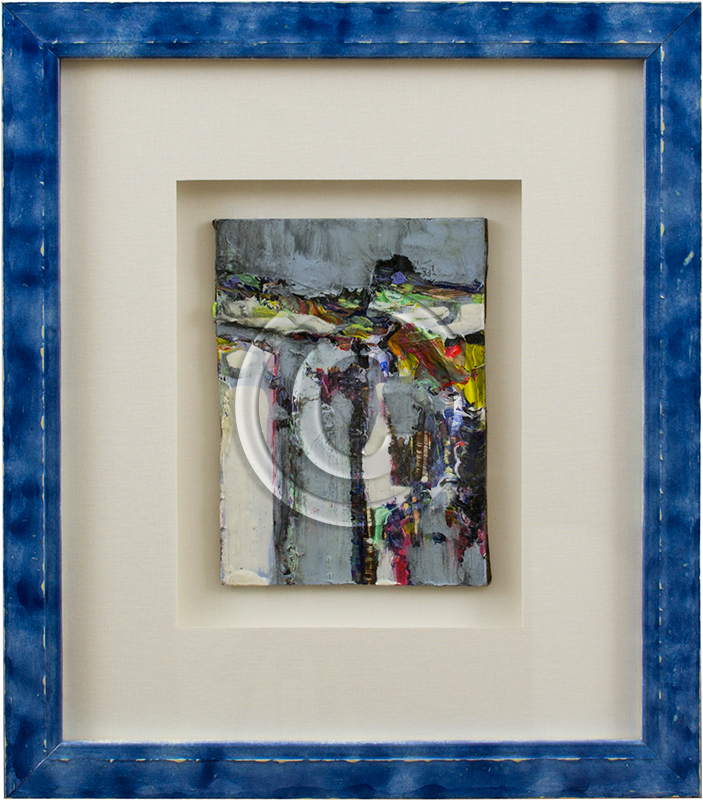This vertical rectangular image features a framed piece of abstract artwork. The distinctive outer frame is predominantly blue, with a gradient blending dark and light shades, suggesting it may have been hand-brushed with acrylics. Surrounding the artwork is a double layer of matting: the outer matting is a cream color, while the inner matting is a slightly deeper beige. 

The abstract painting itself, occupying a smaller central space, features a background that is mostly a lighter blue with splashes of various colors, including yellow, dark blue, red, and orange. Key elements within the painting include a couple of white circles, with one circle nested within another, suggesting a target-like shape. Additionally, there's a prominent vertical bar rising from the bottom, intersected by two horizontal bars extending from either side. The chaotic yet intentional composition features a variety of shapes and colors, which creates a visual complexity that is both intriguing and aesthetically appealing.